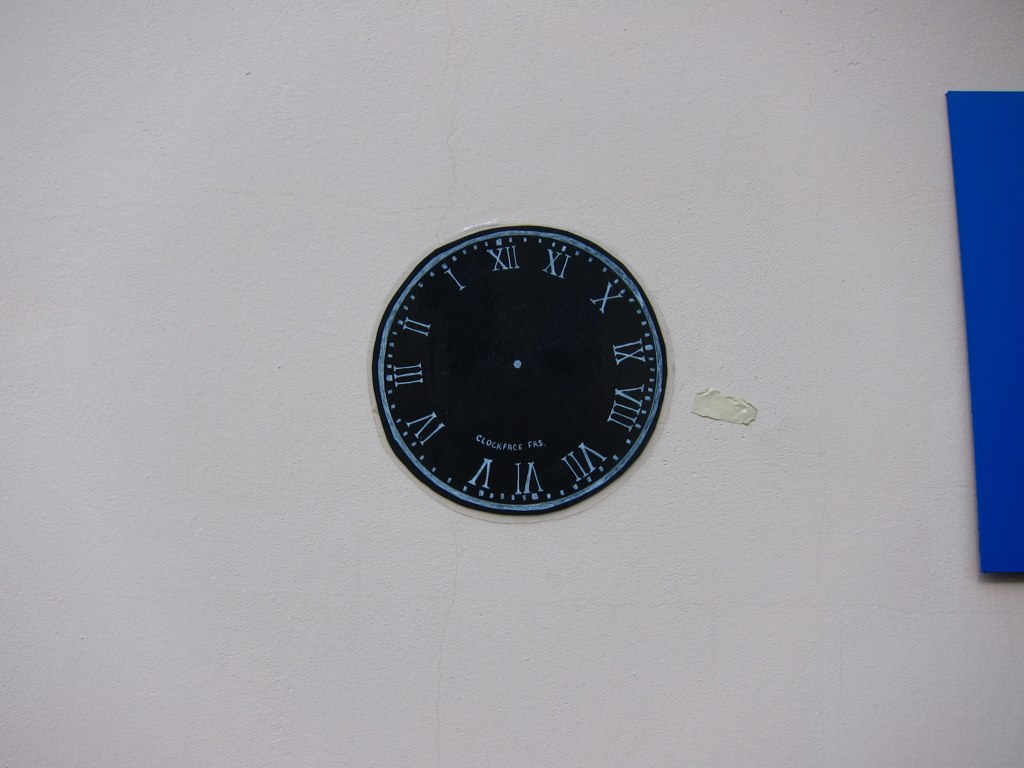This detailed photograph captures a unique black clock against a white plaster wall. The clock appears to be molded or painted directly onto the wall, lacking a traditional case and hands. Roman numerals in white border the face, distinctly running counterclockwise: starting from 12 at the top left and progressing down numerically through 11, 10, and so on. The clock's alignment is slightly off-center, with the number 12 just to the left of the vertical top. At the bottom of the clock face, small text reads "Clock Face FKS." Additionally, there is a patch of white tape or plaster filling a hole beside the clock. To the right of the clock, there is a partially visible royal blue square affixed to the wall, featuring a thin blue line that extends downwards, adding a subtle contrast to the otherwise monochromatic setting.